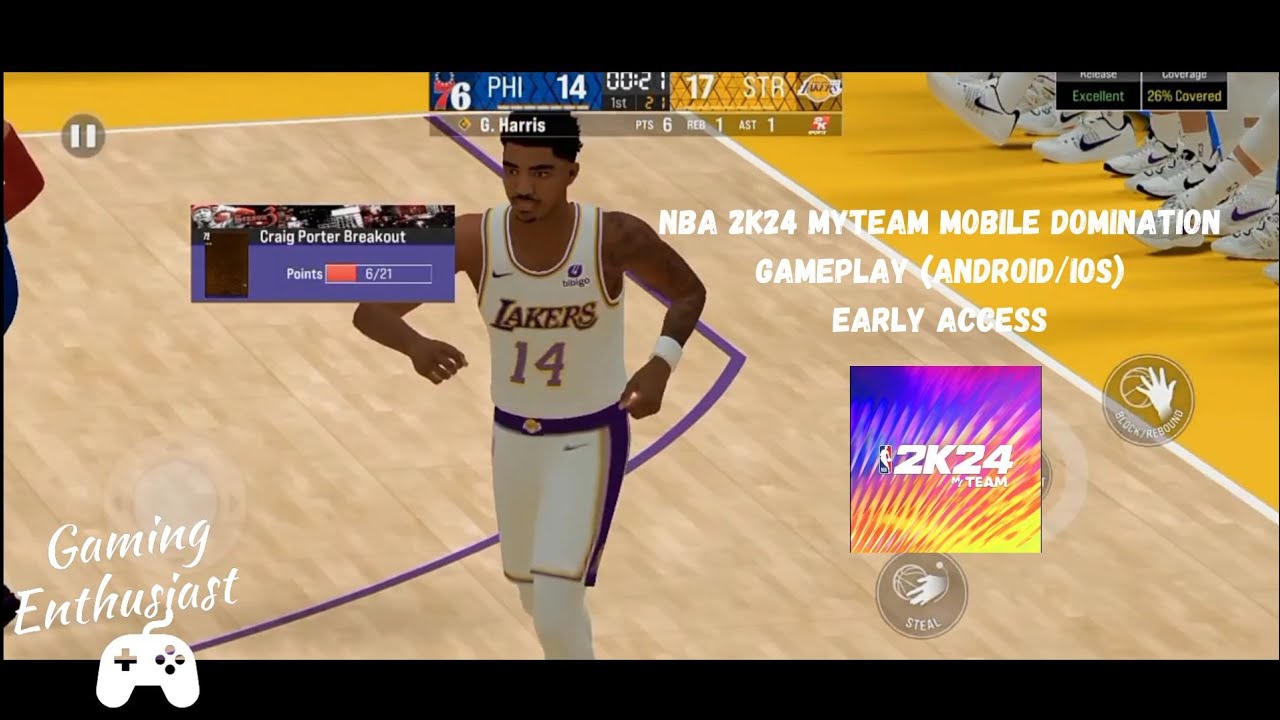In this detailed screenshot taken from the NBA 2K24 video game, you can see a character prominently positioned in the center, running towards the viewer with a slight inclination to the left. The character is dressed in a white Lakers jersey, marked with the name "Lakers" and the number "14" on the chest. Above the gameplay scene, the scoreboard displays the current score, with Philadelphia at 14 points and the Los Angeles Lakers leading with 17 points. 

On the right side of the image, text reads "NBA 2K24 My Team Mobile Domination Gameplay, Android, Early Access," accompanied by a link for the game NBA 2K24, suggesting an early access feature on mobile platforms. Additionally, the bottom left-hand corner features a logo with the words "Gaming Enthusiast" in white text, situated above a white video game controller icon. This comprehensive scene highlights the immersive and competitive nature of the virtual basketball game.